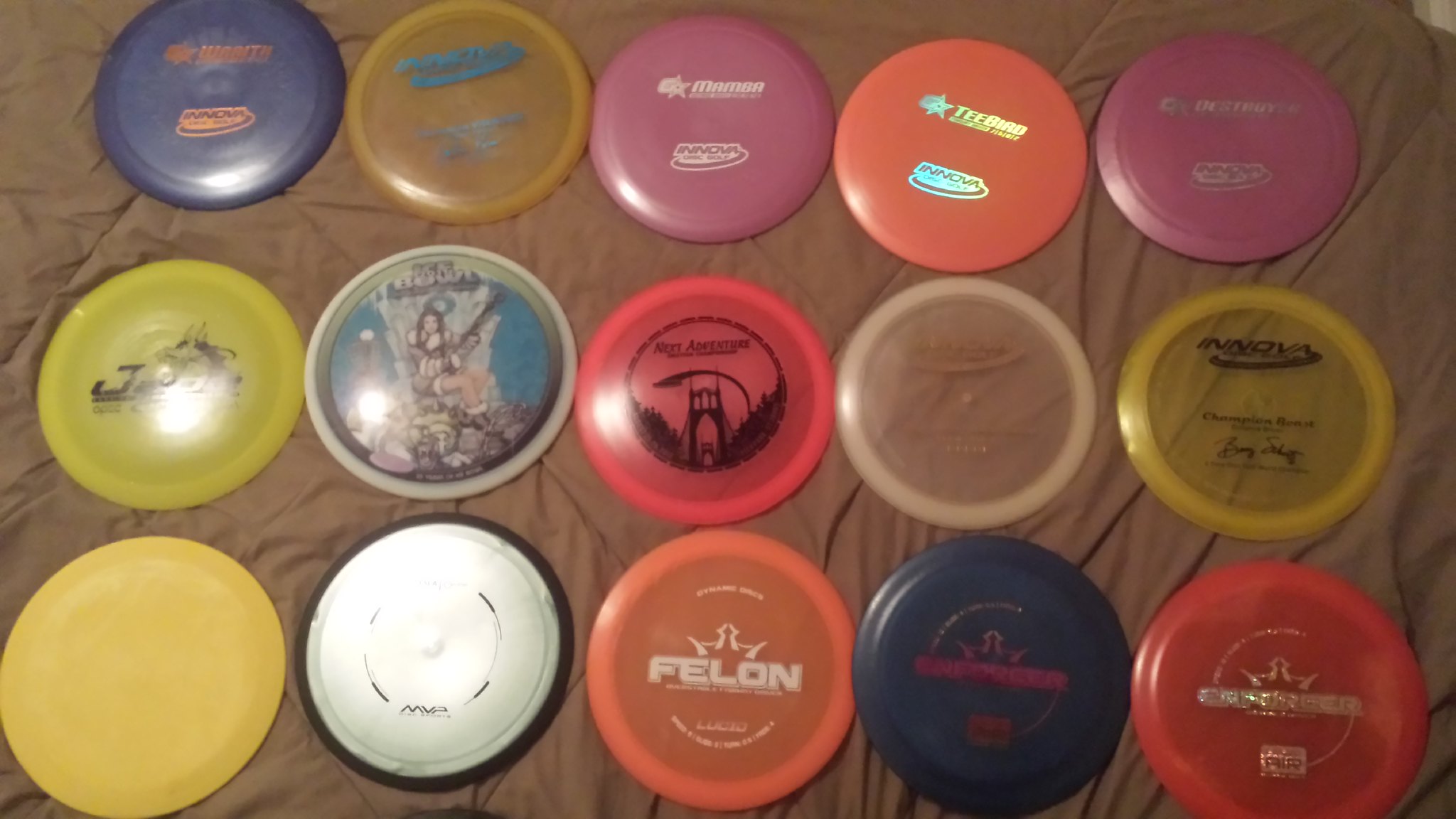This is a detailed color photograph of fifteen plastic discs, which appear to be frisbees, arranged neatly on a tan piece of cloth. The discs are organized into three rows of five. Each disc is unique in color and design, adding a vibrant and eclectic feel to the composition. In the first row, the sequence progresses from blue, yellow, pink, orange, to dark pink. The second row features a yellow disc, a blue disc with a drawing of a young woman, followed by a red disc, a clear disc, and another yellow disc which is transparent. The bottom row displays a yellow disc, a white disc with a black rim, an orange disc with the word 'felon' printed in white lettering, a black disc, and a red disc. The condition of the discs varies, with some showing signs of wear where the writing has been partially scratched off, while others appear newer with more legible markings. The overall scene is set against a medium-brown sheet or bed covering, which acts as a neutral background to highlight the diverse colors and designs of the frisbees.